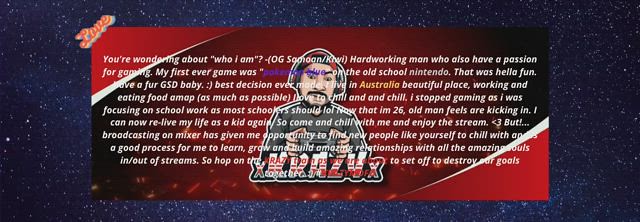The image features a narrow, horizontally aligned rectangular banner with a dark blue space background filled with tiny white stars. At the center is another horizontal rectangle shaded in red at the upper left and lower right corners, fading to a darker red in between. This central rectangle contains a paragraph of white text partially obscured by an animated image of a man with a black mustache and wearing a hat. The text introduces him as an "OG Samoan Kiwi," a hardworking man passionate about gaming who fondly remembers his first game on the old-school Nintendo. He shares that he has a German Shepherd dog, lives in Australia, and enjoys working and eating food. He mentions taking a break from gaming to focus on schoolwork and, at the age of 26, looks forward to reliving his childhood by streaming. Inviting others to join his streams on Mixer, he expresses his enthusiasm for building relationships with new people and learning from the streaming community. The text speaks of his desire to grow, have fun, and achieve goals together with his viewers.